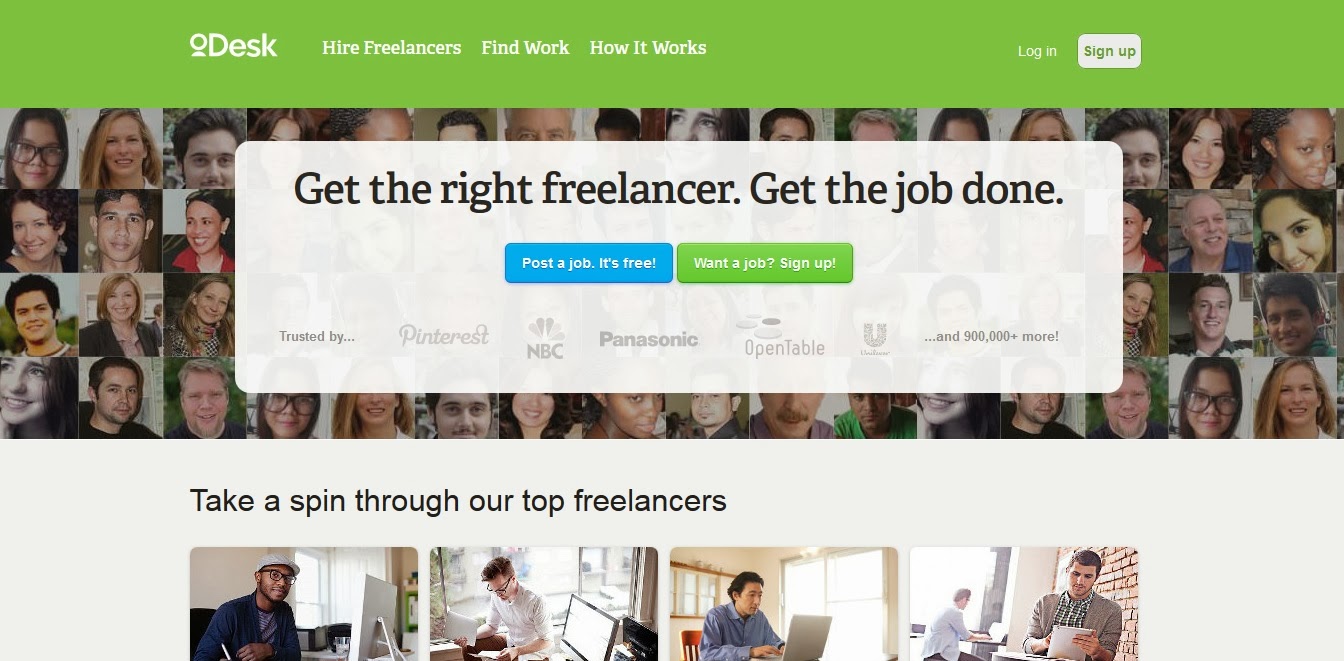In the image, the top section features a green box with white text and a small white icon of a person at a desk. The text includes options such as "Hire Freelancers," "Find Work," "How it Works," "Log In," and a "Sign Up" button. Below this, a large central image showcases a collage of approximately 30 to 40 photos of various freelancers. 

In the middle of this large image, there is a prominent white block with the words "Get the right freelancer, get the job done," followed by a blue button labeled "Post a Job – It's Free" and a green button labeled "Want a Job? Sign Up." 

At the bottom of this section, there are logos of companies like Pinterest, NBC, Panasonic, Pinnable, and others. Below that, a light blue box features the text "Take a spin through our top freelancers" alongside images of four individuals working at their desks on computers.